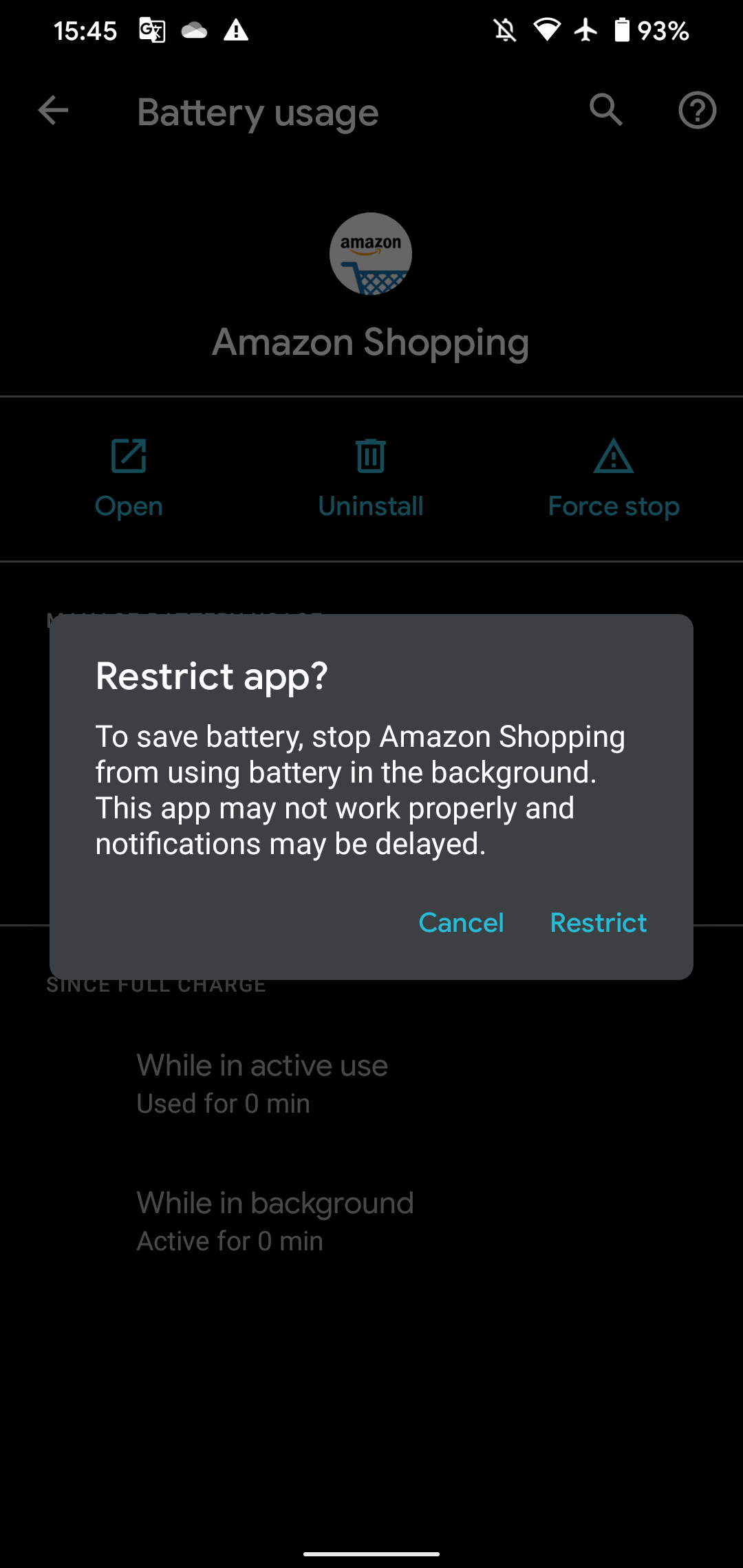**Detailed Descriptive Caption:**

This image depicts a screenshot taken from a mobile phone displaying the battery usage interface. In the top left corner of the screenshot, the time is shown as 3:45 PM. There are three notifications visible at the top: one from Google Translate, another likely related to cloud storage, and a caution notification with an exclamation mark inside a triangle. In the top right corner, icons indicate that notification sounds are disabled, Wi-Fi is connected, airplane mode is on, and the battery is charged to 93%.

The main focus of the screenshot is the "Battery usage" page for the Amazon Shopping app, identifiable by its logo and app name displayed at the top of the screen. Below the app name, three options are available: "Open", "Uninstall", and "Force stop". A central pop-up notification says, "Restrict app to save battery," explaining that restricting the Amazon Shopping app will prevent it from using battery power in the background, though it may impact the app's performance and the timeliness of notifications. This pop-up offers two actions in blue text: "Cancel" or "Restrict."

The user appears to have chosen the "Restrict" option, prompting this confirmation message. Beneath this pop-up, obscured text is visible with sections labeled "While in active use" and "While in background." It states that the Amazon Shopping app has used zero minutes in both active use and background activity.